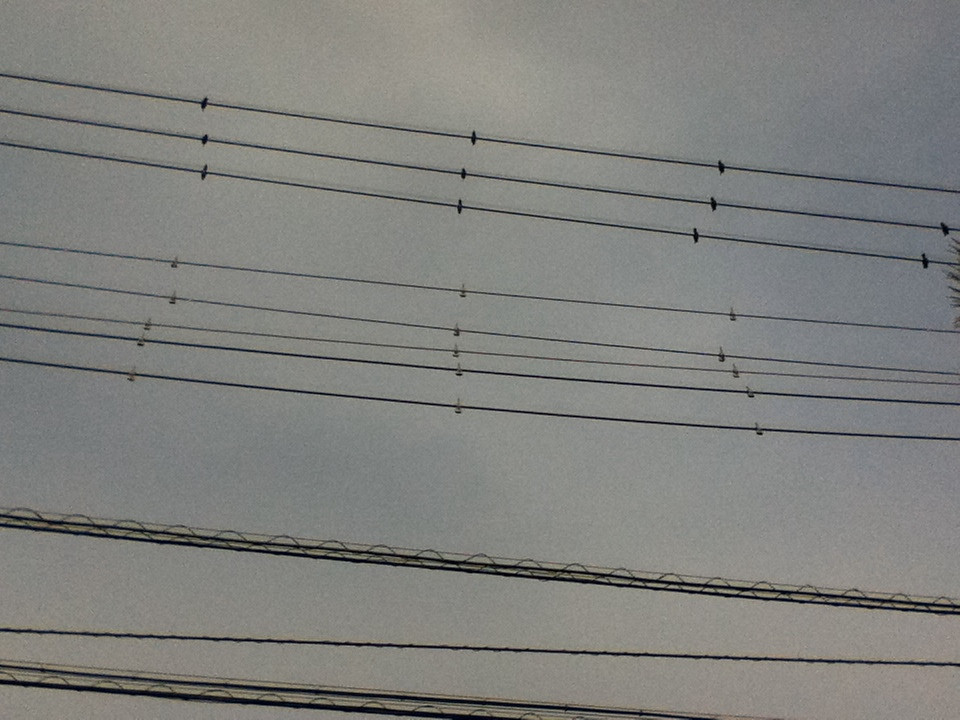This amateur, low-quality photograph captures an overcast sky with just a hint of blue, featuring a series of black power lines set diagonally across the gray, barely blue-tinted backdrop. There are a total of 10 power lines in the image, divided into three distinct groups. The top section consists of three lines, each segmented by small metallic nodes that appear almost like perched birds. Just below, there are five more wires with similar but less evenly spaced nodes. Near the bottom of the image, there are two thicker lines, each interwoven with a coiled wire. Off to the mid-right edge of the photograph, the tips of what appears to be tree branches or some sort of plant are faintly visible, adding a natural element to the otherwise industrial scene. The sky and power lines dominate the frame, with no text, date stamp, or description to provide context.